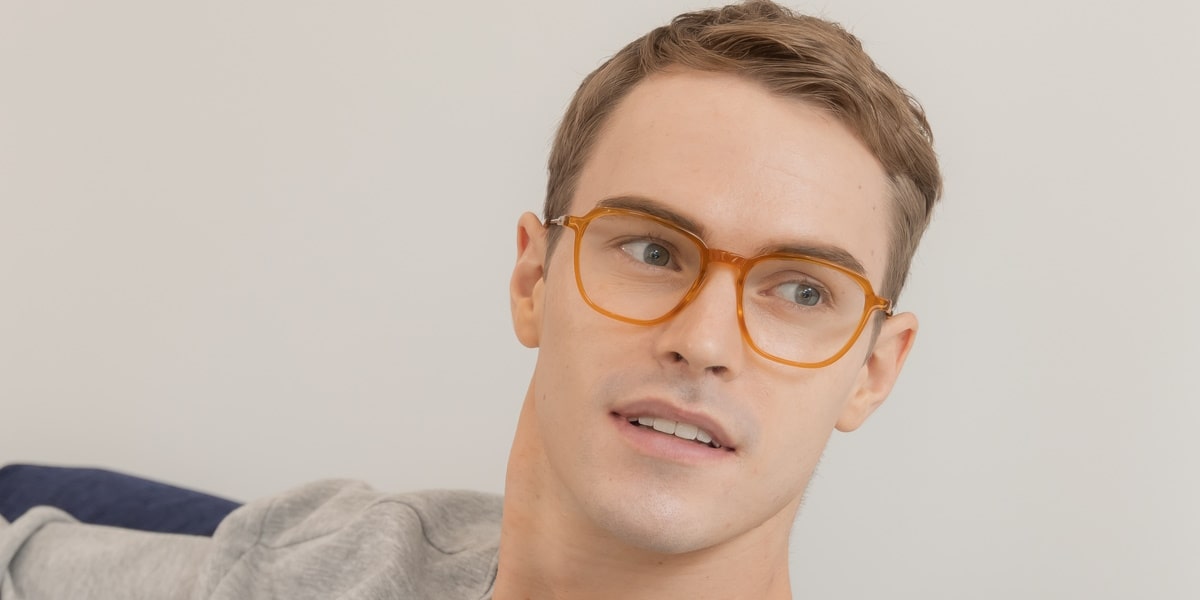This is a detailed photograph of a young white man in his 20s, shot indoors. His head is slightly tilted to the right, showcasing his green eyes and neatly groomed short brown hair. Wearing distinctive orange or brown translucent glasses, his expression is relaxed with his mouth slightly open, revealing straight white teeth. He has the beginnings of a mustache, creating a faint shadow above his upper lip. His attire is casual—a gray sweatshirt, part of which is visible along with his shoulder and a portion of his arm. The setting features a light-colored wall and the edge of a blue sofa or chair on the left side of the image, with this blue object enhancing the cozy ambiance of the room. The overall composition centers his face with a clear, sharp focus, hinting at a model-like poise.